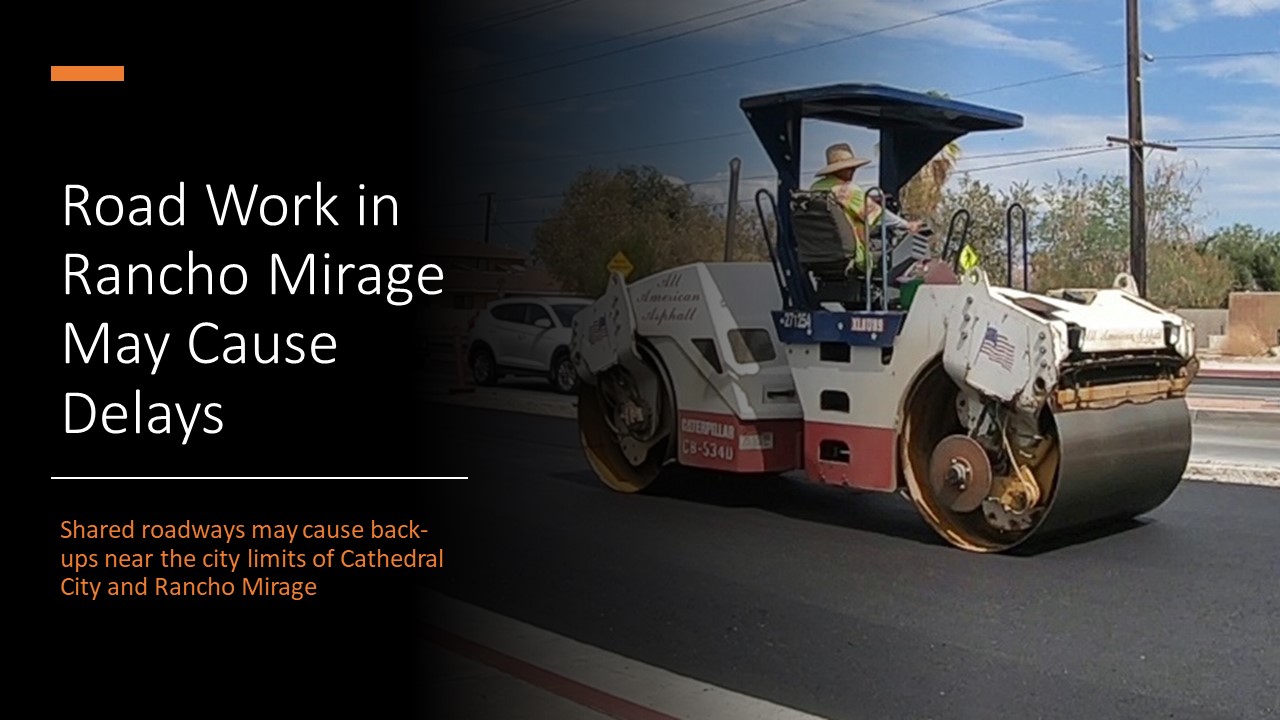A detailed color photograph functions as a Public Service Announcement (PSA), alerting residents of Rancho Mirage and Cathedral City, California, about imminent road maintenance. Against a partly cloudy sky with visible telephone poles and a white truck in the backdrop, a man operates a white and red steamroller on freshly paved asphalt. He dons a straw hat and a neon green and orange safety jacket, focusing intently on his task. Positioned to the left of the image, an orange bar and a black gradient block background transition seamlessly into the photo. Large white text announces, "Roadwork in Rancho Mirage may cause delays," and smaller orange text underneath warns, "Shared roadways may cause backups near the city limits of Cathedral City and Rancho Mirage." The composition and clear sky suggest a sunny day as the message effectively informs locals about potential traffic disruptions due to ongoing construction work.